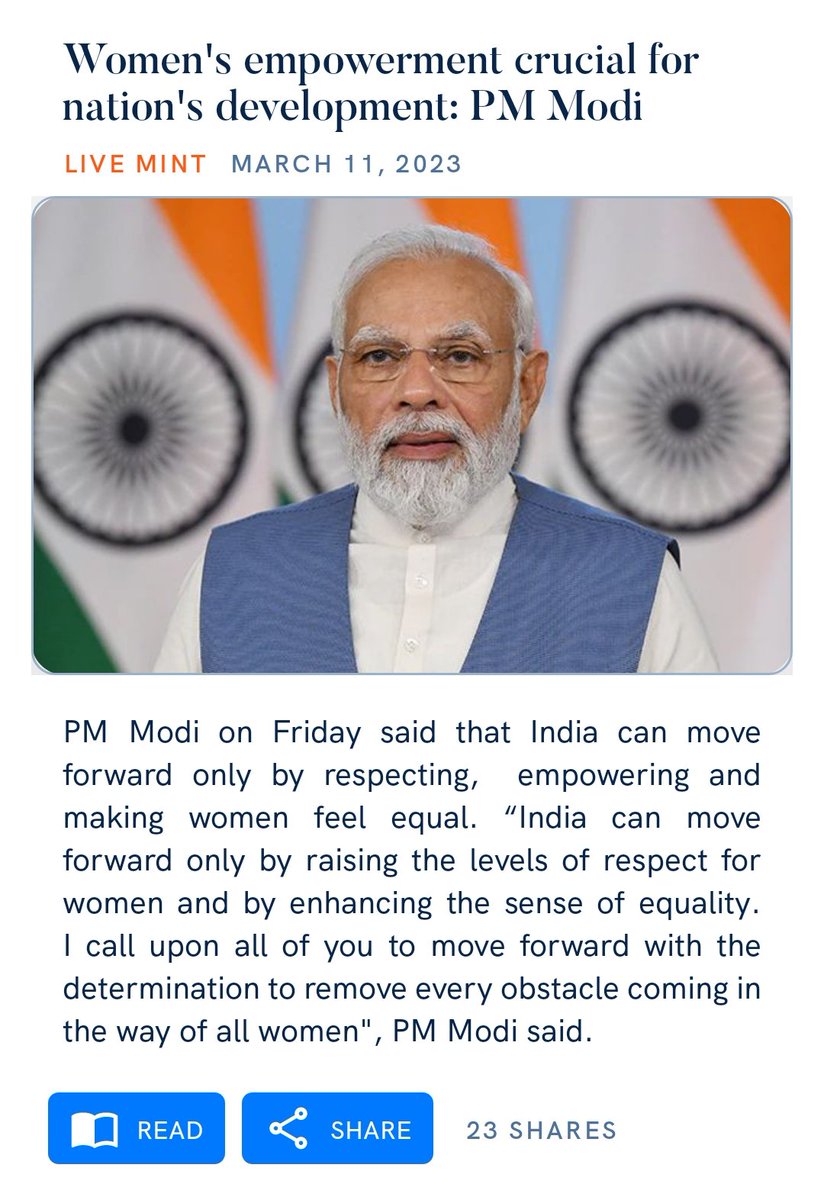Here is a cleaned-up and detailed descriptive caption for the screenshot:

---

The screenshot depicts an article excerpt from the blog LiveMint, with the header "LiveMint" prominently displayed at the top in bold black letters. The article headline, "Women's Empowerment Crucial for Nation's Development: PM Modi," is positioned just below in large text. To the left of the headline, "LiveMint" is repeated in bold red capital letters, and to the right is the date, "March 11th, 2023," in large gray font.

Beneath these elements is a substantial thumbnail image of Prime Minister Narendra Modi. An excerpt from the article follows, quoting PM Modi's statement made on a Friday, emphasizing the essential role of women's empowerment in India’s progress. The quote highlights the necessity of respecting, empowering, and ensuring equality for women. He calls on the public to commit to eliminating obstacles that hinder women's progress.

At the lower section of the screenshot, there is a blue "Read" button and a "Share" button. Adjacent to the share button, it indicates that the article has been shared 23 times, shown in smaller gray text.

---